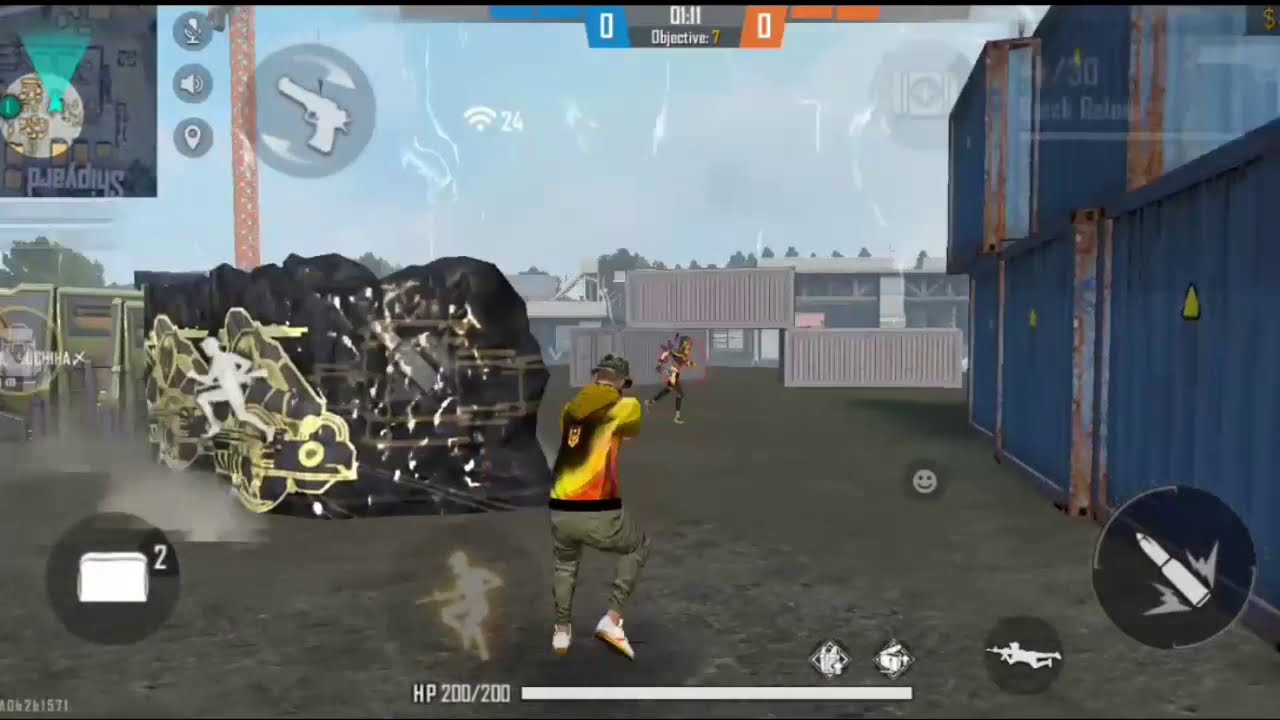The image depicts a still from a video game featuring a dynamic scene with two characters engaged in combat. One character, dressed in dark green cargo pants, white sneakers, and a distinctive black, yellow, and mustard sweatshirt, is aiming a gun at a target in the distance. This character is wearing a bucket hat and is positioned to the left of the frame. The other character appears to be running away, heading towards the right side of the image. The backdrop suggests a junkyard or industrial area with various blue, rusted storage containers and a white fence visible. Close to the shooter, there seems to be a parked motorcycle or a similar vehicle.

Overlaying the scene is a scoreboard at the top of the image, displaying a score of 0-0 for both the blue and orange teams, indicating a tie. The timestamp at 01:11 suggests that the game is still in its early stages. Additionally, the HUD shows the player's health at a full 200 out of 200 and indicates that the current objective is marked with the number 7. The detailed environment and character attire suggest the players are participating in a high-stakes, multiplayer match, navigating through a gritty, equipment-laden battlefield.